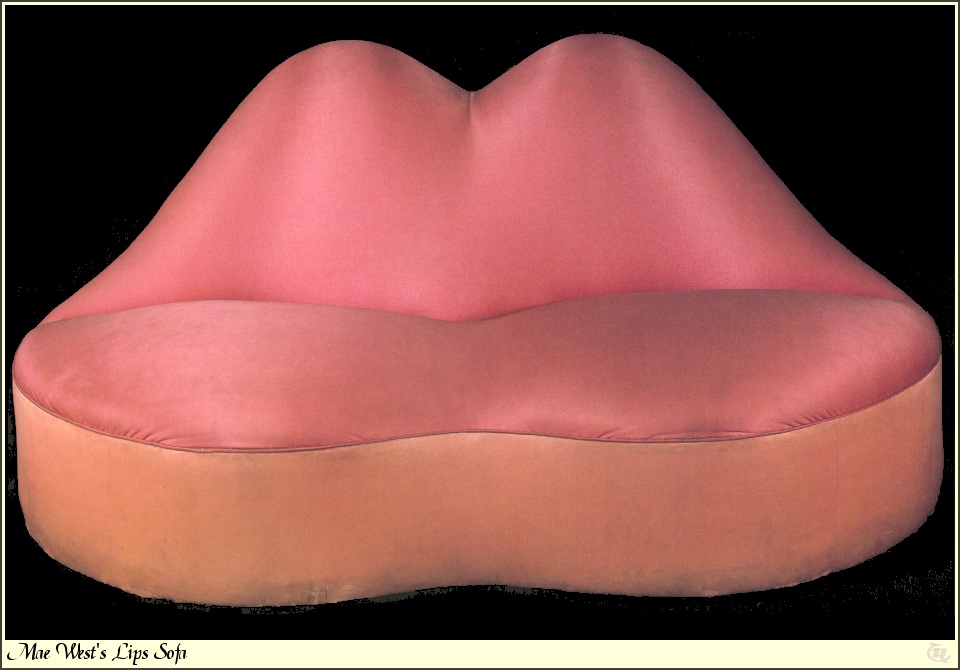The image presents a detailed and close-up photograph of a distinctive pink sofa designed to resemble human lips, famously known as the "Mae West Lip Sofa." Set against an entirely black background, this striking piece of furniture is centrally positioned, taking up most of the image. The sofa’s unique design features the seat forming the bottom lip and the backrest forming the top lip, both crafted with a shiny, glossy cloth that enhances its vibrant pink color. The bottom edge of the sofa is bordered with a peach orange or tannish-yellow hue. The text "Mae West Lip Sofa" is visible at the bottom of the image, lending to its artistic appeal and confirming its iconic design. There are no other objects present in the photo, emphasizing the sofa's prominence, making it appear as if it could be an eye-catching advertisement for a luxury furniture website.